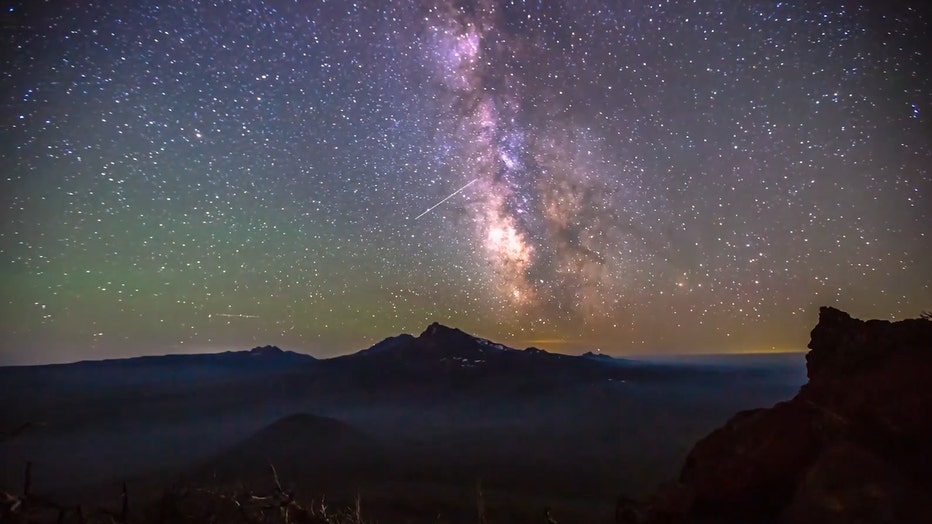A stunning nighttime photograph capturing a vast, star-filled sky over a serene desert landscape. The bottom third of the image is draped in darkness, punctuated by a rugged hill on the right. To the right of the hill, a prominent rocky outcrop stands out against the dark backdrop. In the distance, a gentle range of mountains peeks up, their silhouettes barely discernible.

The night sky above is a spectacle of countless tiny stars, scattered like cosmic confetti across the heavens. Dominating the center of the photograph, slightly to the right of the mountain peak, is a bright, radiant light. From this focal point, a segment of the Milky Way stretches upwards, creating a cloudy band that fades to darker tones on the right. The left part of the Milky Way band is brighter, and through it, a diagonal streak of light ascends into the middle of the image, adding an element of dynamic movement to the scene.

Just above the horizon, a hint of yellow light glimmers faintly where the sky meets the earth, perhaps a lingering trace of sunset or distant artificial light, gently illuminating the edge of this breathtaking nocturnal landscape.